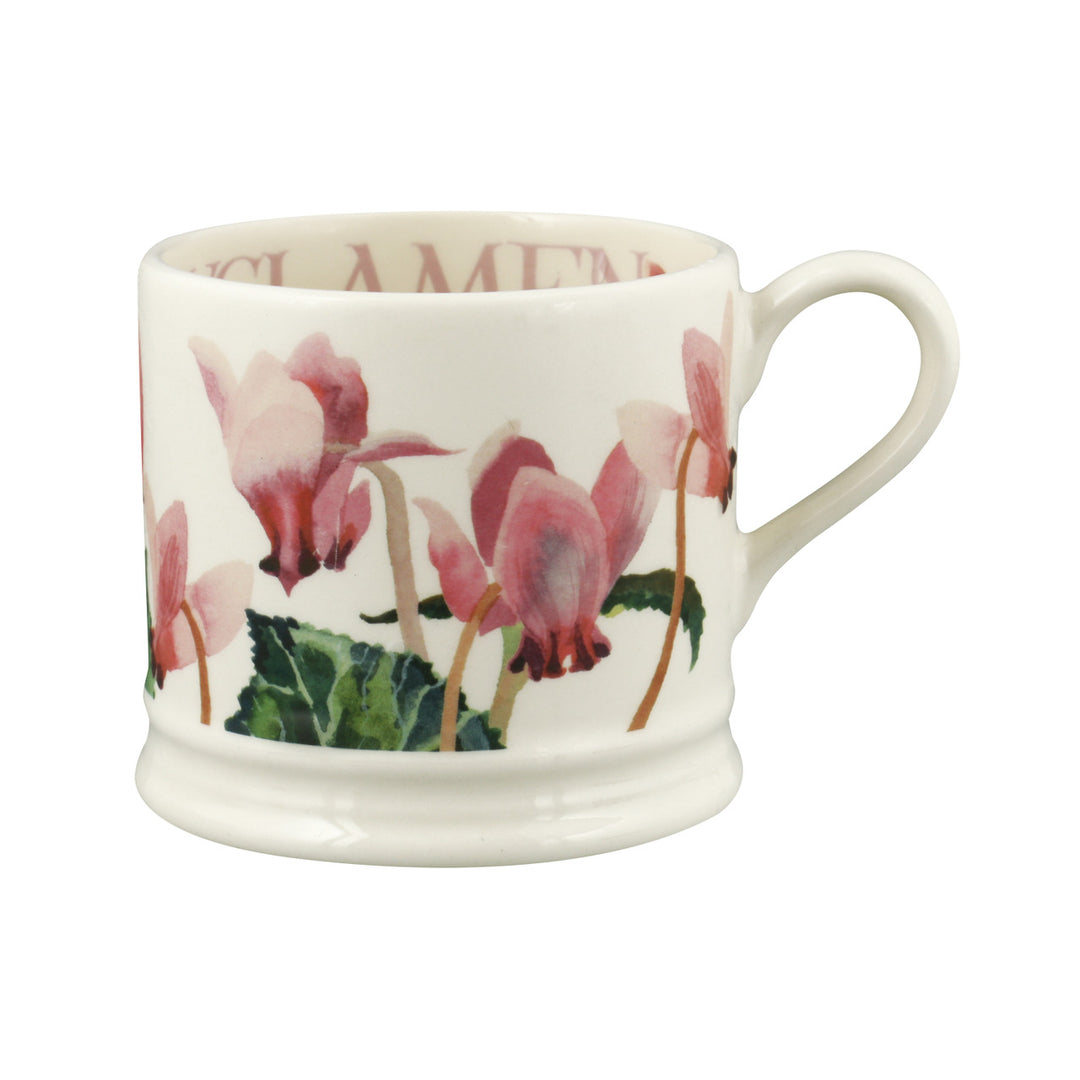This is an image of a predominantly white ceramic mug, featuring a design that includes stems with pink flowers and green leaves. The flowers, each with slightly varied shades of pink petals, appear unique but belong to the same type. The mug's handle is oriented to the right, suggesting a small opening that might accommodate one or two fingers. The base of the mug flares out slightly, likely for added stability. Inside the mug, there are partially visible words that suggest letters like 'A', 'M', 'E' or 'F', and 'N,' with the text appearing to be in pink. Rocking a flat and unique design, this mug stands out for its aesthetic appeal.